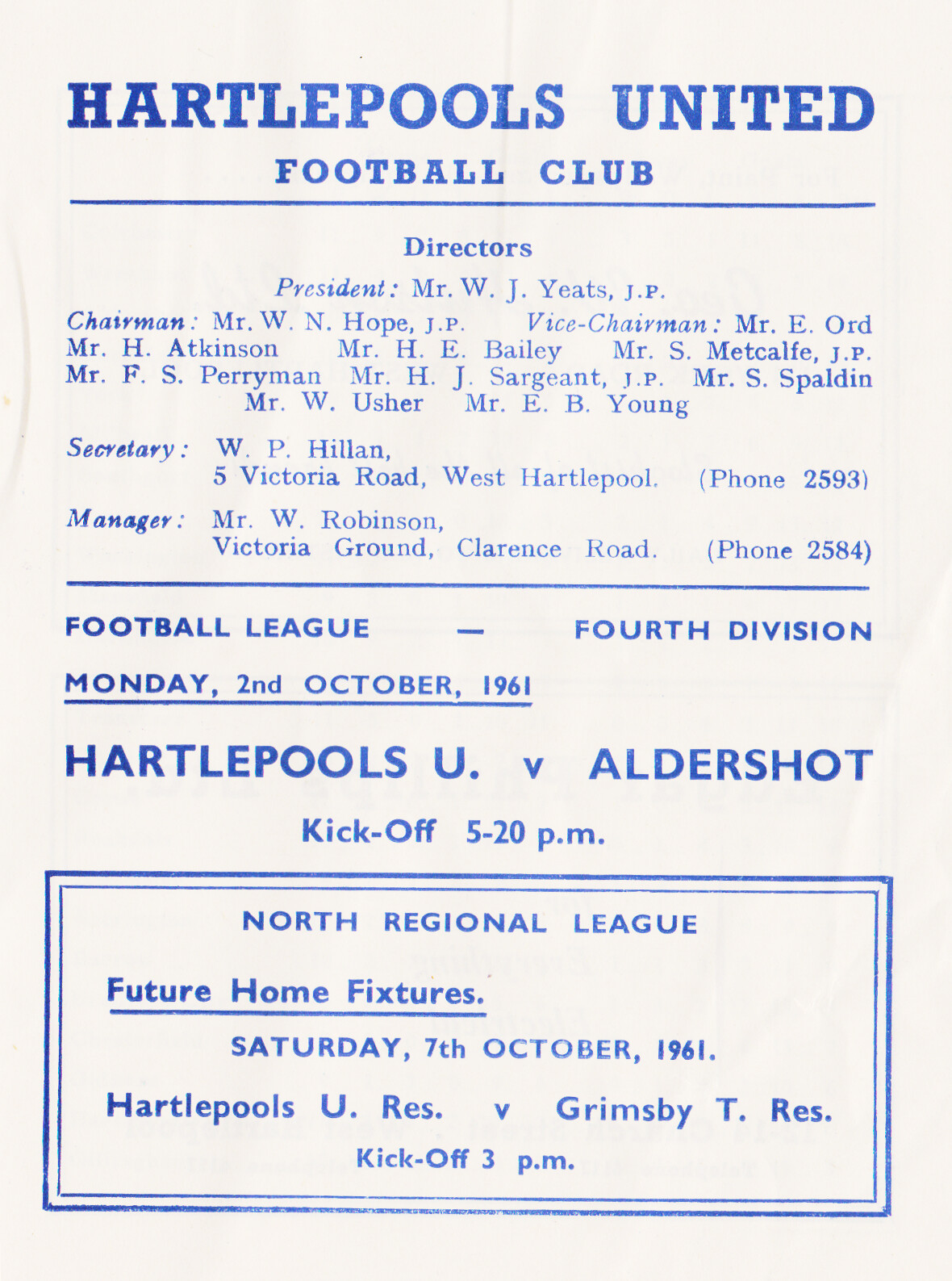The image depicts a slightly wrinkled white piece of paper with all-blue lettering, resembling the front page of a football program or advertisement. At the top, it prominently features "Hartlepools United Football Club" in all caps. Below a thin blue dividing line, it lists key officials including President Mr. W.J. Yeats, J.P., Chairman Mr. W.N. Hope, J.P., Vice Chairman Mr. E. Ord, and several directors such as Mr. H. Atkinson and Mr. S. Metcalf, J.P. The Secretary is listed as W.P. Hillen, 5 Victoria Road, West Hartlepool, phone 2593, and the Manager is Mr. W. Robinson, Victoria Ground, Clarence Road, phone 2584.

Another blue line separates this section from the next, which notes the date "Monday, 2nd October 1961," and the match details "Hartlepools U versus Aldershot, kickoff 5.20pm" in larger text. At the bottom, enclosed in a blue rectangle, are details for the North Regional League future home fixtures, specifying "Saturday, 7th October 1961, Hartlepools U-Res versus Grimsby T-Res, kickoff 3pm."